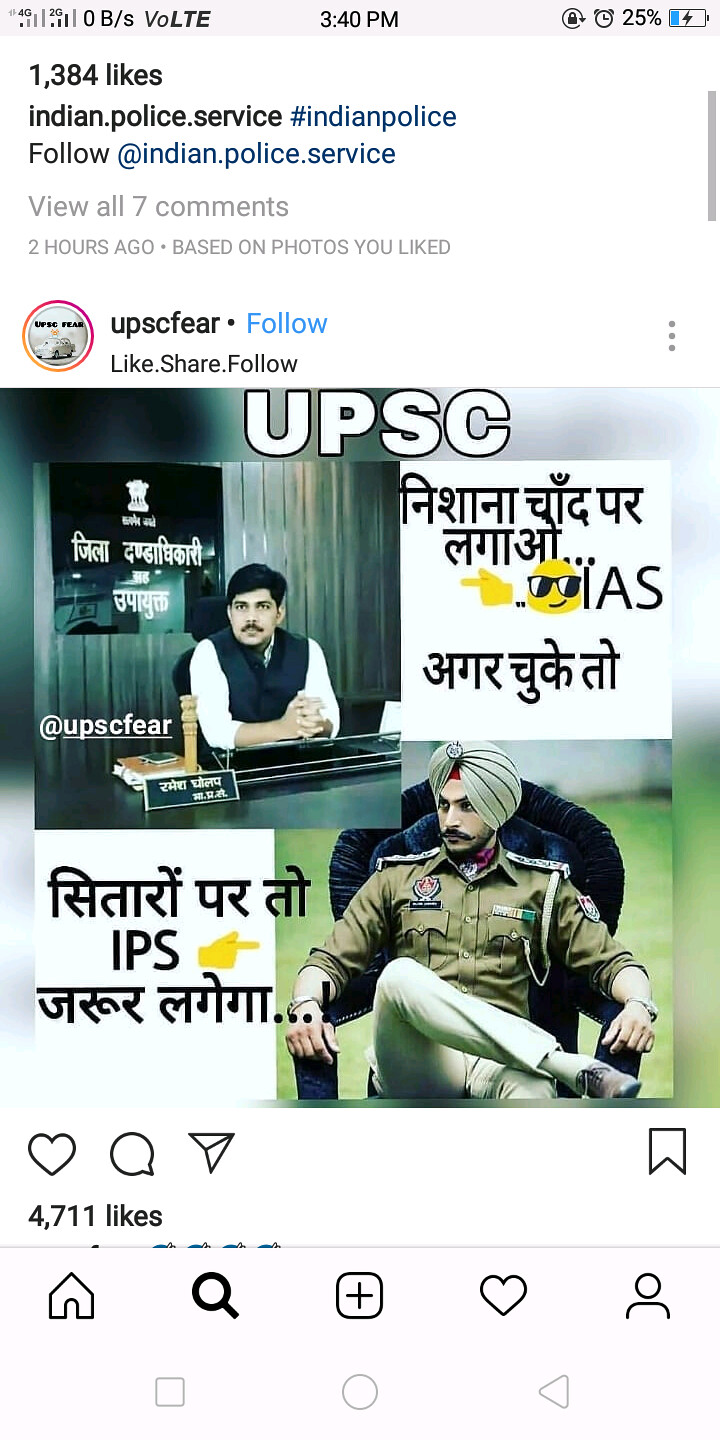The image depicts a screenshot from what appears to be a social media feed, likely Instagram, displayed on a mobile phone interface. The top bar of the phone screen shows indicators such as 4G reception, a timestamp reading 3:40 p.m., an alarm clock symbol, and the battery life at 25%. The post has amassed 1,384 likes and seven comments and is associated with the Indian Police Service, with mentions to follow the UPSC Fear account. At the center of the post, there is a photograph featuring two Indian men. The man sitting in a chair is dressed in a military-style uniform with distinguishing insignia, suggesting a high-ranking position, and is wearing a turban. The second man is positioned behind a clerk's desk, looking serious. The image is accompanied by text in Hindi and contains promotional elements encouraging users to like, share, and follow the account.